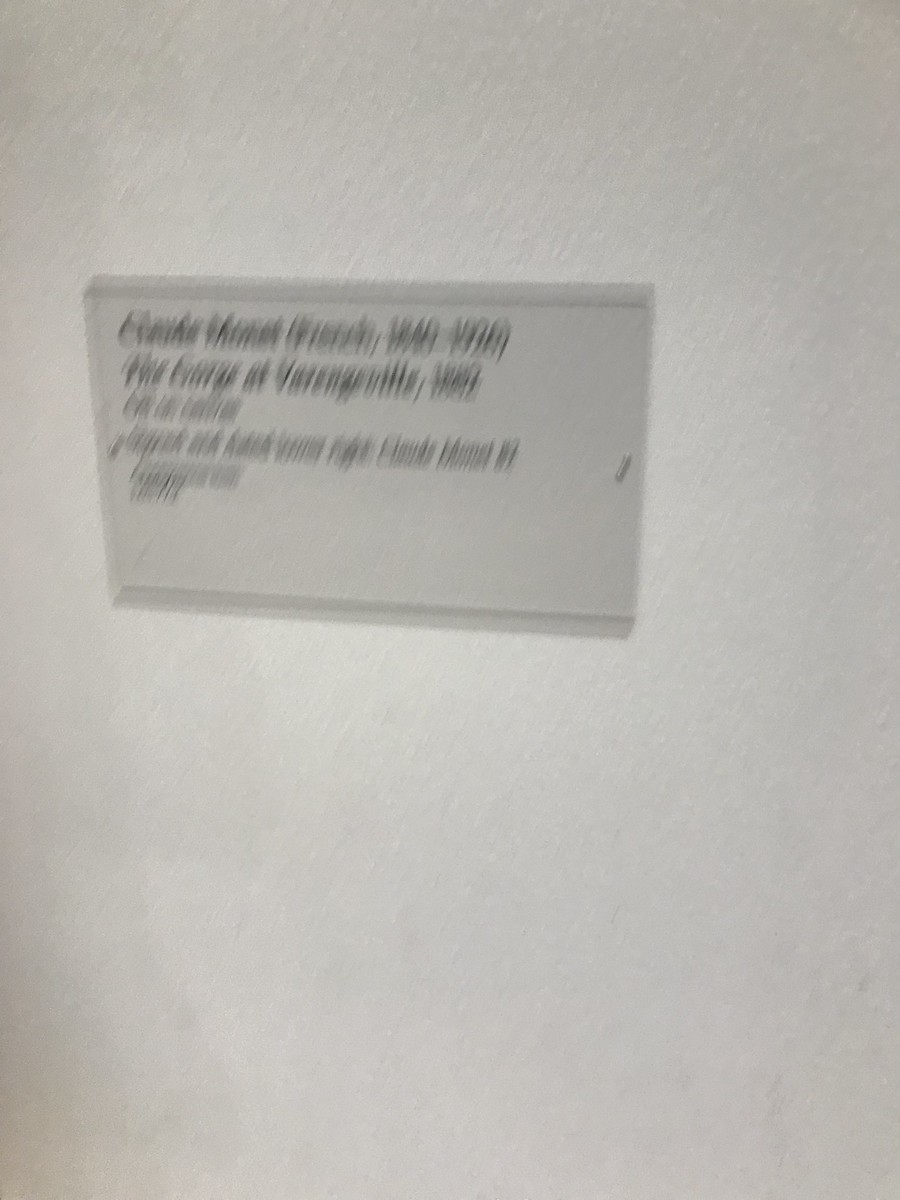The image showcases a pristine white wall adorned with a distinctively labeled artwork by Claude Monet, believed to have been created in 1926. The focal point is an elegant placard, providing pertinent information about the piece. The placard appears to be made of glass with printed text, possibly detailing the title and number associated with the artwork. This glass placard is affixed to the wall using two delicate screws, one on the left and one on the right, subtly blending in and almost unnoticeable unless closely examined. The overall setting exudes a sense of quiet reverence, emphasizing the importance and delicate nature of the displayed piece.